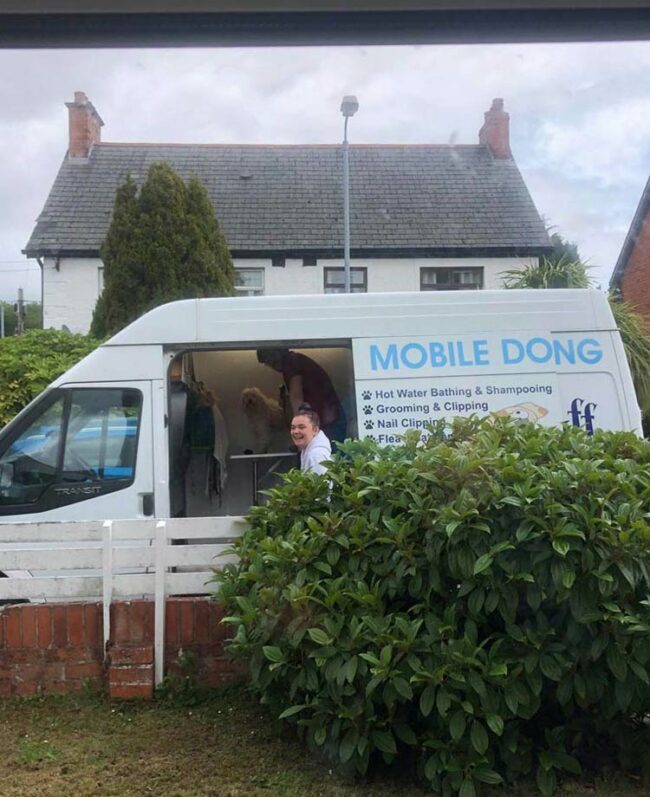In this outdoor photograph, we see a large white van parked on the road in front of a white house and a white picket fence that sits atop a wall made of brown bricks. To the right, a big green shrub partially obscures the van. The van door is open, revealing the interior where a dog is being groomed on a table. A woman wearing a white hoodie stands at the edge of the van, smiling. A man, who appears to be in a red shirt and blue pants, is in the back of the van. The van has light blue text on the side, but the open door overlaps with some of the text, humorously altering "Mobile Dog Grooming" to "Mobile Dong." Below that, more text reads: "Hot Water Bathing and Shampooing, Grooming, Clipping, Nail Clipping," though it is partially obscured by the shrub. The setting appears to be in a suburban area with a cloudy grey sky overhead.